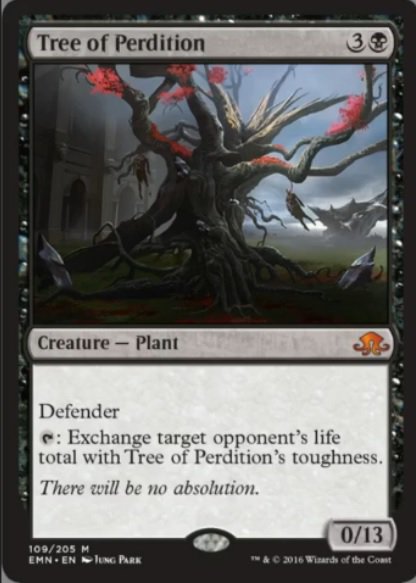The image is a detailed screenshot from a card game, showcasing an intricately designed playing card set against a black background. The card, predominantly dark in tone, features a sinister and towering tree known as the "Tree of Perdition." The edges of the card are adorned with elaborate designs framing the central image and text.

At the very top of the card, a long horizontal light brown bar bears the name "Tree of Perdition" in black text. Adjacent to the name, there are two small circles: one displaying the number "3," and the other featuring a tiny black skull, indicating the card's mana cost. 

The main illustration depicts a large, menacing black tree with gnarled roots jutting out from the ground. The tree appears to be in the process of ensnaring a person on the left side, while a fiery aura of red flames emanates from its upper branches. In the backdrop, a stormy sky looms ominously, with hints of a castle silhouetted against the tempestuous weather.

Beneath the image, another bar reads "Creature — Plant," next to a small orange icon. The card's special ability is explained in text: "Defender. Exchange target opponent's life total with Tree of Perdition's toughness. There will be no absolution."

In the bottom right corner of the card, a stat box indicates the Tree of Perdition’s power and toughness as "0/13." At the very bottom of the card, there is a small note: "© 2016 Wizards of the Coast," denoting the publisher and date of the card's creation.